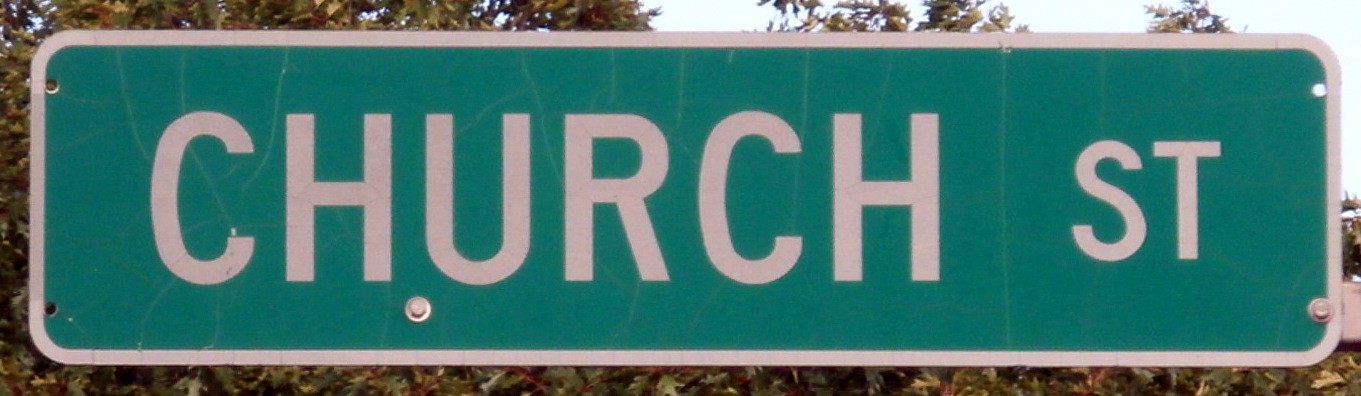This close-up, cropped photograph prominently features a green and white street sign for "Church Street." The rectangular street sign, which nearly fills the entire frame, is bordered with a white edge and has rounded corners. Displayed in bold white letters, "Church" is larger and more pronounced than "ST," also rendered in white. The sign has four drilled holes in the corners: two on the left and two on the right, with a single screw securing it at the lower right. Additionally, there is a silver screw positioned between the letters H and U in "Church." The sign's background reveals a mix of brownish-green trees and foliage, with leaves lining the bottom edge of the photo, and glimpses of a white and blue sky peeking through the top and center right.